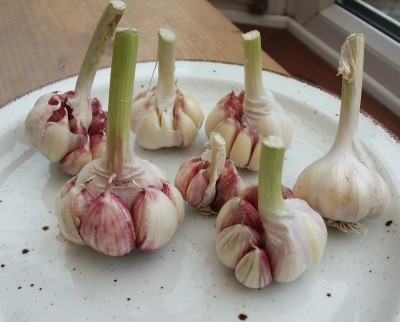The image displays a white, somewhat old-fashioned plate with black and brown spots, suggesting either dirt or a deliberate vintage design. The plate, which takes up most of the frame and extends off the image's edges, rests on a light brown wooden table. Atop the plate are seven garlic bulbs, varying in size and color. Most of the bulbs are full-sized with pink and white cloves, while two are predominantly white with white stems. One smaller, center-positioned bulb is particularly notable for its pink and white hues with a white stem. The garlic stalks exhibit a range of colors from slightly green to dried-out white. Scattered around the bulbs are brown and black specks, potentially remnants from freshly harvested garden garlic. In the background, beyond the table, part of a red or burgundy floor and a white-bordered area, possibly a wall or window, are faintly visible, adding context to the setting.